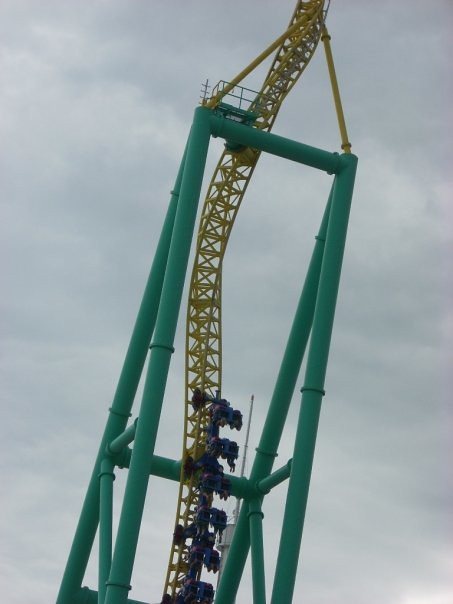The photograph, taken during daytime under a cloudy gray sky, captures a thrilling roller coaster in action. The image features a towering yellow track that twists and spirals downward, supported by a robust green pipe-like scaffold framework. The scaffolding consists of large green cylindrical metal bars with multiple cross beams, forming a sturdy triangular structure. At the heart of this intricate setup, a single yellow track snakes through the green framework, starting from a platform and descending in dramatic loops. The roller coaster itself is comprised of free-floating blue chairs without bottoms, allowing the riders' feet to dangle freely in the air as they experience the exhilarating descent. This snapshot vividly portrays both the architectural complexity and the electrifying motion of the ride.